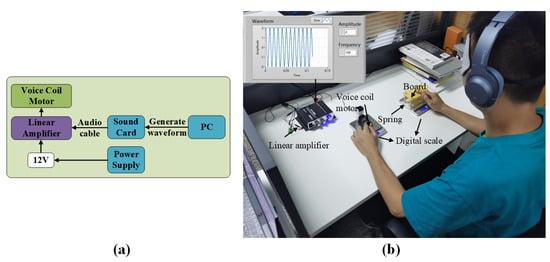The image is composed of two main parts. On the left side, labeled "Picture A," there is a green rectangle bordered in black, containing a detailed diagram. The diagram illustrates the setup for a sound creation and monitoring system. It includes several elements: from a "PC" generating a waveform going to a "Sound Card," which then connects via an "Audio Cable" to a "Linear Amplifier." The "Linear Amplifier" is linked to a "Voice Coil Motor." Additionally, a "Power Supply" (indicated by a teal rectangle) provides 12 volts of power, connecting to the same "Linear Amplifier."

On the right side, labeled "Picture B," there's an image of a man with short black hair, wearing headphones, seemingly assembling the components detailed in the diagram. He is seated at a desk with numerous labeled parts laid out before him, including "Spring," "Board," "Digital Scale," "Linear Amplifier," and "Voice Coil Motor." The man appears to be blindfolded. Above him, a gray screen displays sound waves, perhaps monitoring his progress. To his right, several books are spread out on the desk, possibly containing additional instructions or references for the assembly process. The overall scene reflects a meticulous and carefully guided procedure to construct a sound-generating device as per the instructions in the diagram.